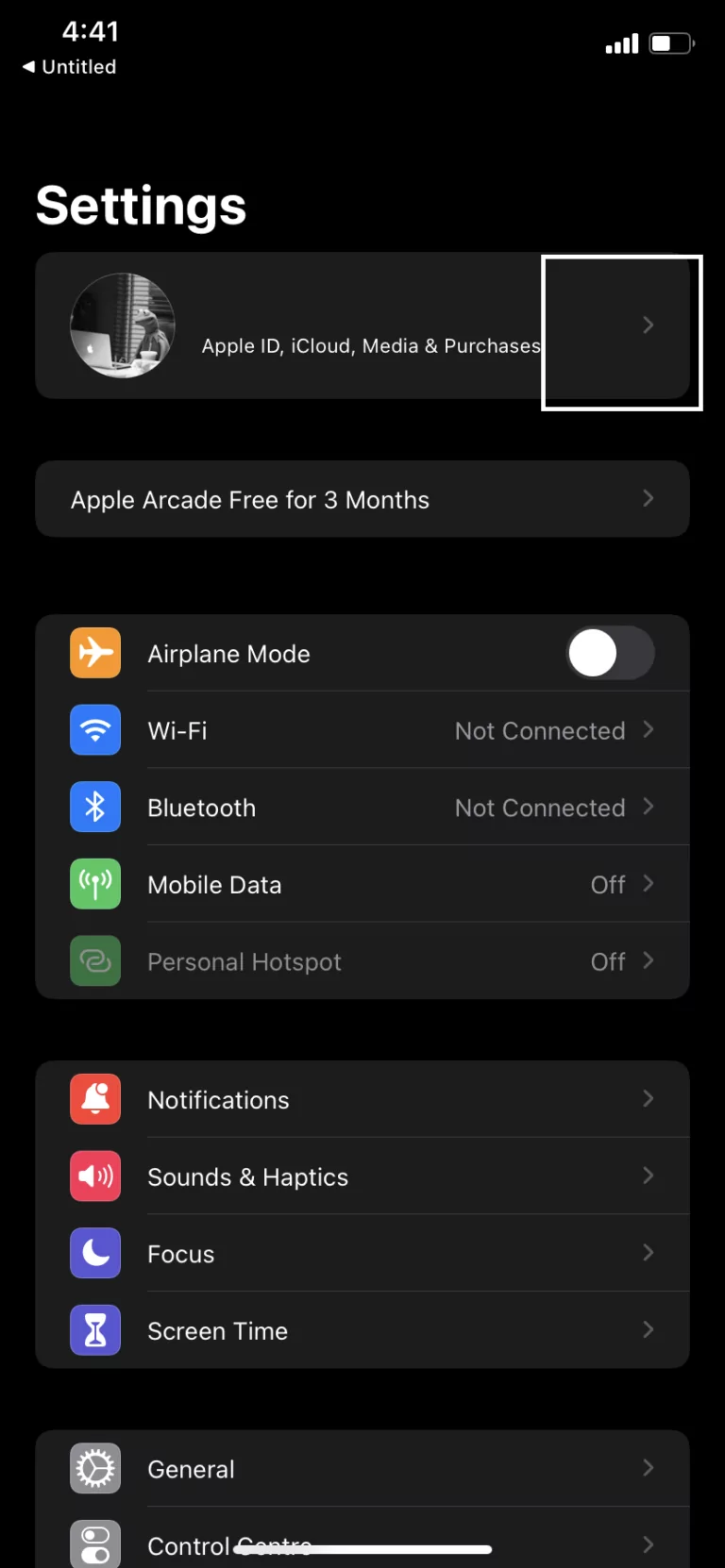The image showcases a settings menu on an Apple device with a sleek black background and crisp white text for readability. At the top left corner, there is a heading that says "Settings". Directly below this, a gray profile icon is prominently displayed, labeled "Apple ID, iCloud, Media, and Purchases". Adjacent to the profile icon on the right side, there is a white square shaded with black, containing a black arrow.

Following the profile section, there is a promotional banner stating "Apple Arcade Free for three months". Below this promotion, a list of settings and apps is displayed. The first setting, "Airplane Mode", features an orange and white icon and is currently toggled off. It is followed by:

- "Wi-Fi", which is not connected, represented by a blue and white icon.
- "Bluetooth", also not connected, indicated with a blue and white icon.
- "Mobile Data", turned off, shown with a green and white icon.
- "Personal Hotspot", switched off, depicted with a green and white icon.

Additional settings include "Notifications", marked by a green and white icon with a white bell; "Sound & Haptics", represented by a pink and white icon; "Focus", displayed with a blue and white icon featuring a moon; and "Screen Time", indicated by a blue and white icon with an hourglass graphic.

At the bottom of the menu, the "General" setting is depicted with a white gear on a gray background, followed lastly by the "Control Center", characterized by a gray and white icon featuring two switch toggles that denote on and off states.